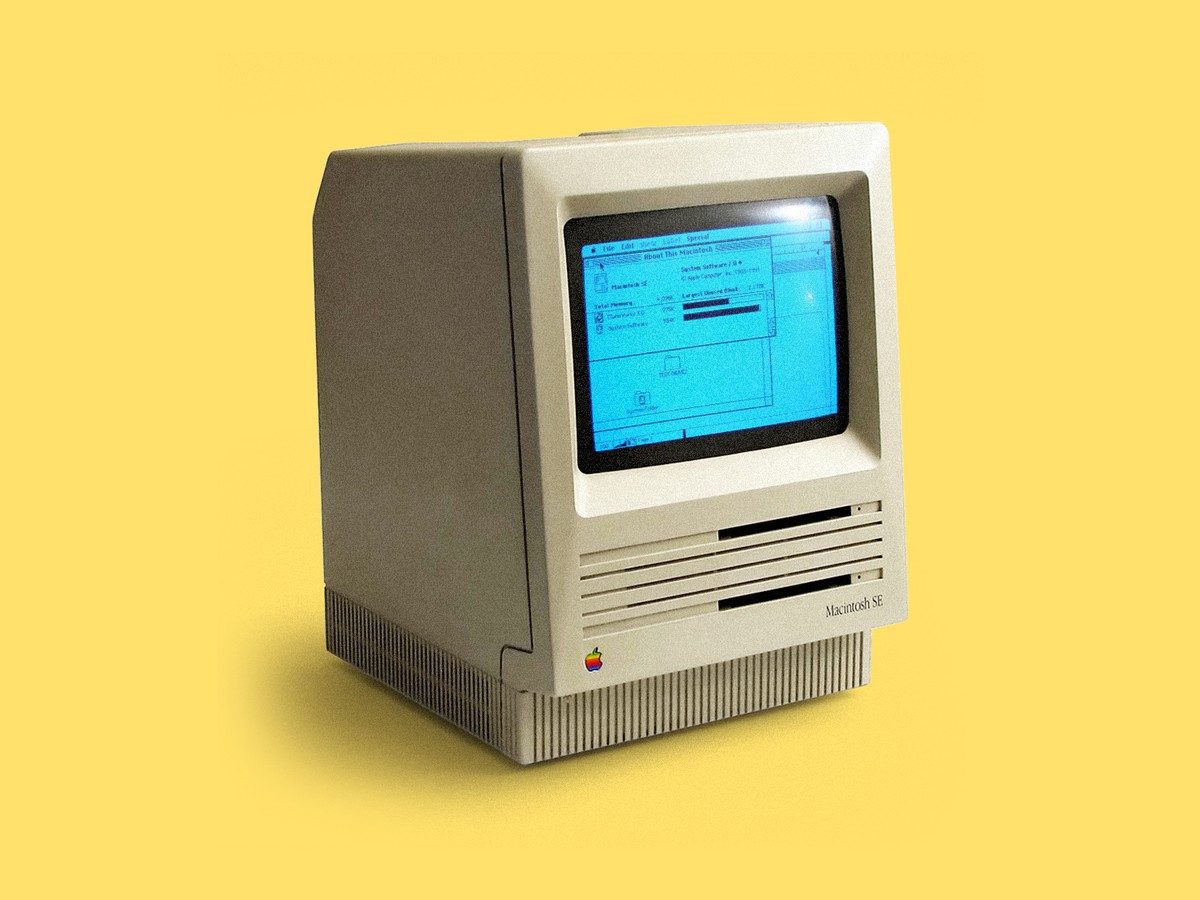This image features a vintage Macintosh SE, one of Apple's early computers from the 1980s. The computer, which is predominantly white, boasts a small, non-high-definition, curved screen that occupies the top half of the front and displays a blurry, angled image with indistinct windows. On the lower left corner of the computer is the iconic Apple logo, represented in its original multicolored, rainbow-striped form. Adjacent to the logo, the model designation "Macintosh SE" is visible. The front panel of the computer features various vertical slits for ventilation, as well as grooves and slots designed for floppy disks. Adding a vibrant touch, the background of the image is a solid yellow color, enhancing the nostalgic feel of this well-maintained relic.